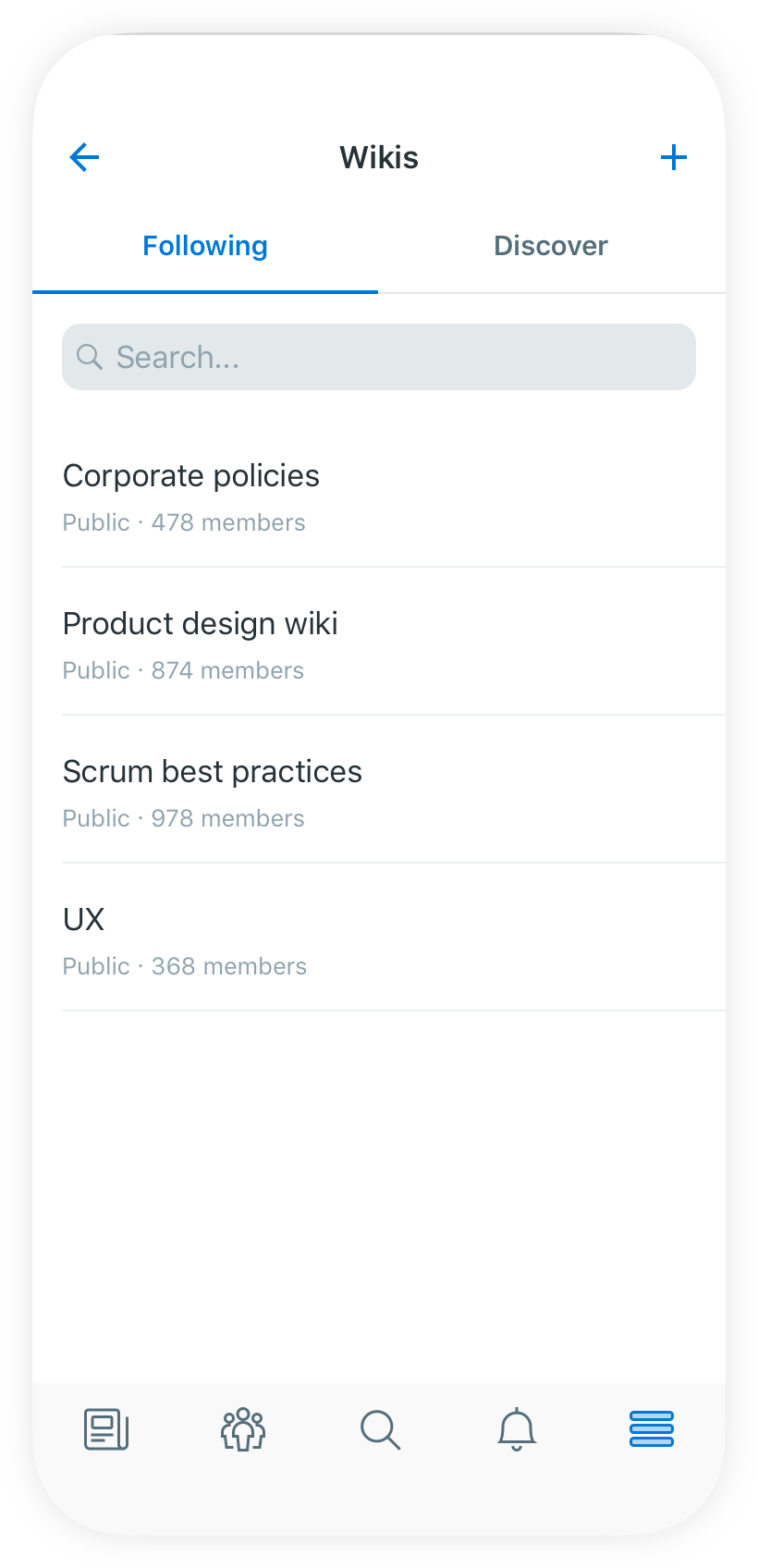The image is a screen capture of a smartphone displaying a wiki management app. At the top of the screen, the title "Wikis" is clearly shown. Beneath it, there's a tab titled "Following" which is highlighted, indicating it is currently selected, while another tab named "Discover" remains unselected. 

Directly under the tabs is a search bar for user convenience. The main portion of the screen includes a detailed list of available wikis, each labeled as public along with their respective membership counts. The entries are:
1. "Corporate Policies" with 478 members.
2. "Product Design Wiki" with 874 members.
3. "Scrum Best Practices" with 978 members.
4. "UX" with 368 members.

All text is presented in black letters on a white background, ensuring readability.

At the bottom of the screen, there is a navigation bar consisting of several stylized icons. From left to right, these icons include:
- An icon that appears to represent a screen with a stylus or a drawing tool, possibly indicating a drawing program.
- An icon showing a group of people, likely representing a community or social feature.
- A question mark, which may lead to a help or FAQ section.
- A magnifying glass for search functionalities.
- A bell icon, commonly used for notifications.
- Three horizontal bars, typically representing a menu or more options.